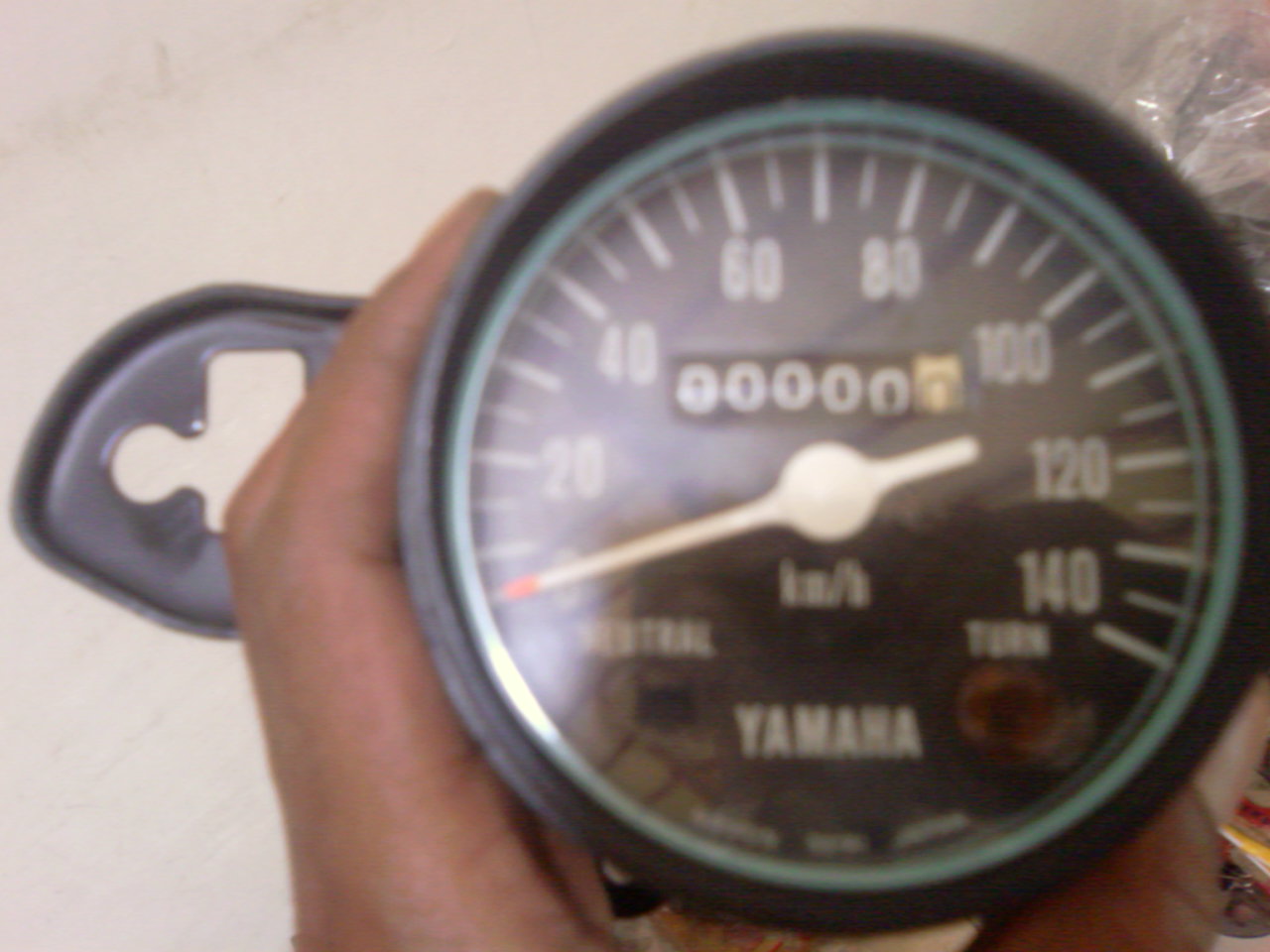In this detailed image, a person is holding a detached speedometer, seemingly from a Yamaha motorcycle. The speedometer features a black outer rim with a silver edge, and its face is black with prominent white numbers and lines indicating speed. At the center, the word "Yamaha" is clearly visible. The speedometer's white needle points towards the gauge, and there's a small odometer window displaying all zeros. The person's thumb is partly visible, situated on the side of the device. Extending from the speedometer's side is a gray projection with a white label shaped like a check stamp. The background reveals a brown wooden table where the speedometer rests. In the top right corner, a plastic bag containing a white object is faintly visible, alongside some small red and yellow items scattered nearby.